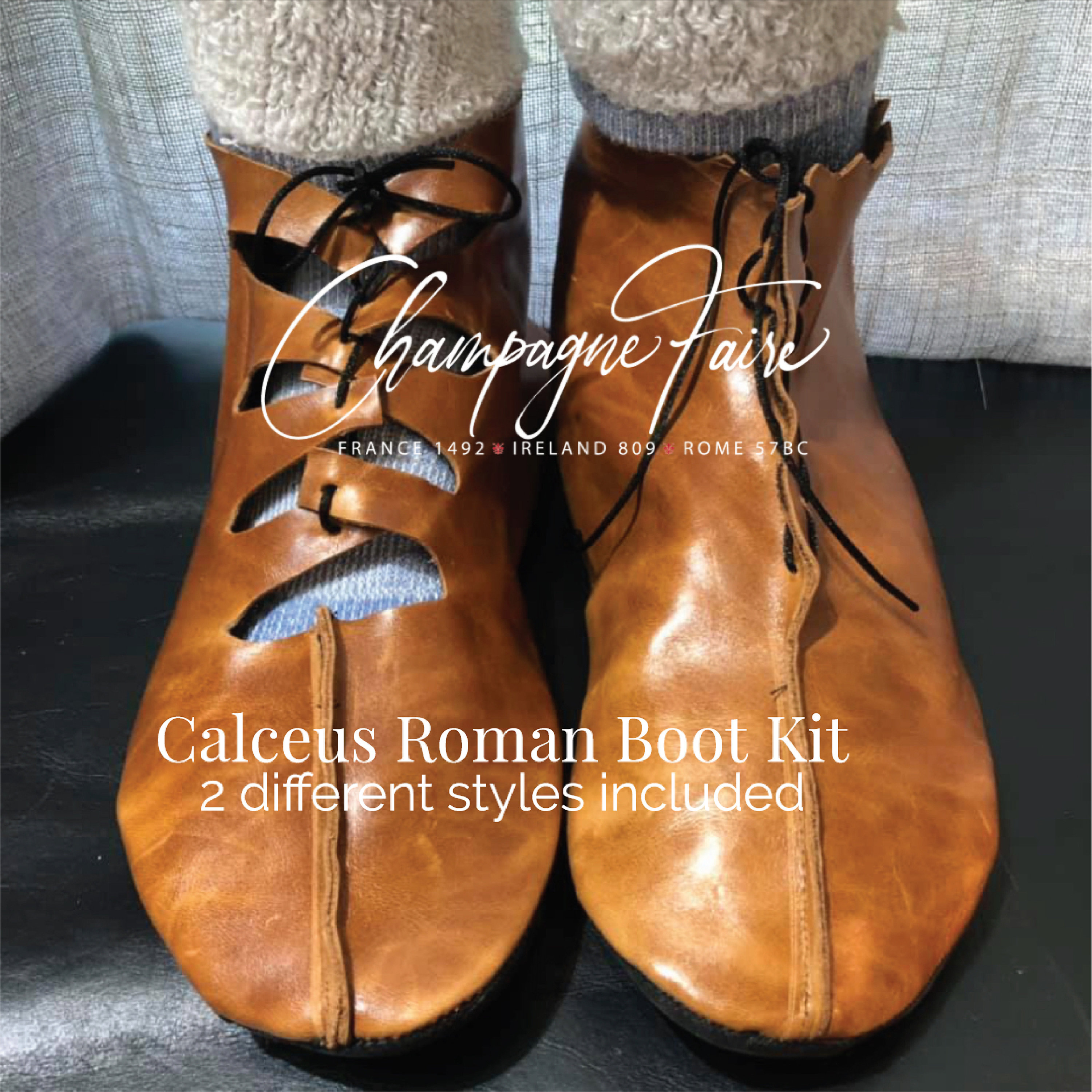This indoor digital photograph showcases a pair of boots with distinct designs, placed against a black backdrop with a thin white curtain behind them. Centered in the image, we see a pair of leather boots, each with different features. The boot on the left has a closed-toe style with black laces running through it, tightening the upper part like that of a modern shoe, revealing purple and blue wool socks worn by the person. The right boot, which appears to be less tightly laced, exposes more of the sock and the inside of the shoe, highlighting the fuzzy wool around the edges. Both boots rest on a black surface, adding contrast to the scene. White text overlays the image, reading: "Champagne Affair France 1492 Ireland 809 Rome 57 BC," followed below by "Calcius Roman Boot Kit, Two Different Styles Included." The predominant colors in the photograph are brown, black, gray, blue, and white.